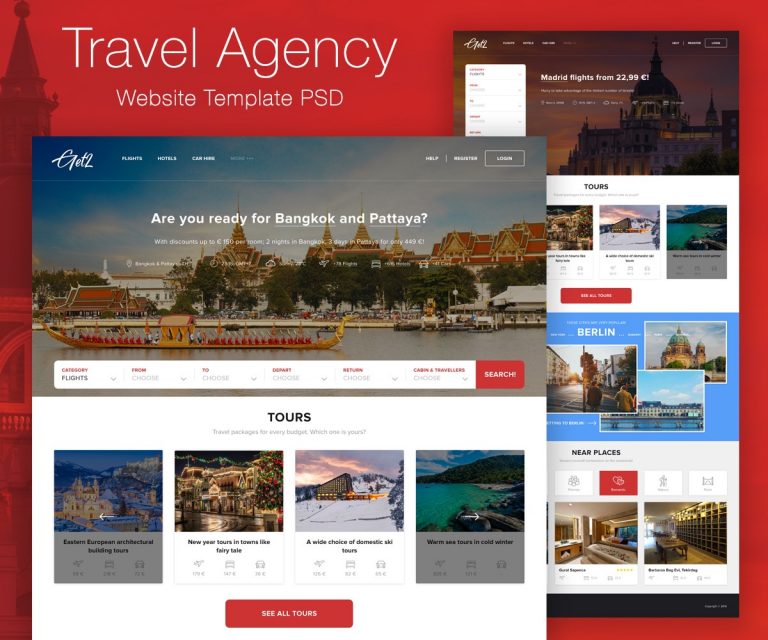Travel Agency Website Template with PSD Design

The image showcases a vibrant travel agency website template, characterized by a striking red border and a prominent header in a matching red hue. At the very top, bold white text reads "Travel Agency," immediately followed by "Website Template PSD" beneath it. 

The main content is divided into two sections:

1. **Highlighted Tours Section:**
   Occupying the lower 70% of the screen, this section features a picturesque scene of Thailand, complete with traditional Thai boats, serene water, temples, and typical housing structures in the background. Overlaid in white lettering is the enticing question, "Are you ready for Bangkok and Pattaya?" This section aims to capture the allure and beauty of Thailand as a travel destination.

   Below this scenic image, there's a white box divided into four smaller boxes, each representing different tour options. Although the exact details of these tours are unclear, there's a clickable button labeled "See All Tours" that invites users to explore further.

2. **Additional Offers Section:**
   Adjacent to the tour highlights, a vertically oriented box draws attention to flights to Madrid, starting from $2299. This section likely offers various tours and hotel options related to Madrid, Berlin, and other nearby places, featuring a list of sites to visit and accommodations, typical of a comprehensive travel agency webpage.

Overall, the template exudes an inviting, professional appeal, designed to captivate potential travelers with its vibrant visuals and organized layout.